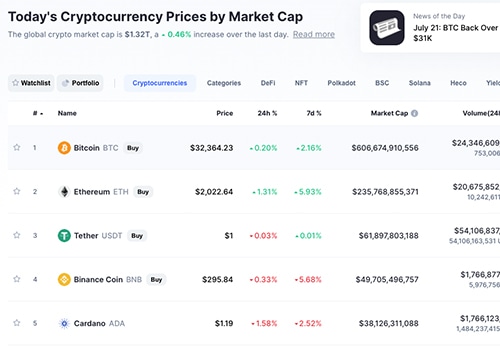This screenshot displays the latest cryptocurrency prices by market capitalization. At the top, it shows that the global crypto market cap is approximately $1.32 trillion, reflecting a 0.46% decrease over the past 24 hours. There's a "Read More" option available for more details.

Beneath this, there's a headline stating, "News of the Day, July 21st: BTC back over 31k." Additionally, the interface includes various sections such as "Watchlist," "Portfolio," "Cryptocurrencies," and "Categories," which serve as filters for the displayed data.

Currently, the top five cryptocurrencies are listed:
1. **Bitcoin (BTC)** - $32,364
2. **Ethereum (ETH)** - $2,022.64
3. **Tether (USDT)** - $1.00
4. **Binance Coin (BNB)** - $295.84
5. **Cardano (ADA)** - $1.19

Each cryptocurrency entry includes details on market cap, 24-hour trading volume, 24-hour price change, and 7-day price change. The screenshot captures only a portion of the list, showing just the top five cryptocurrencies due to limited screen space.